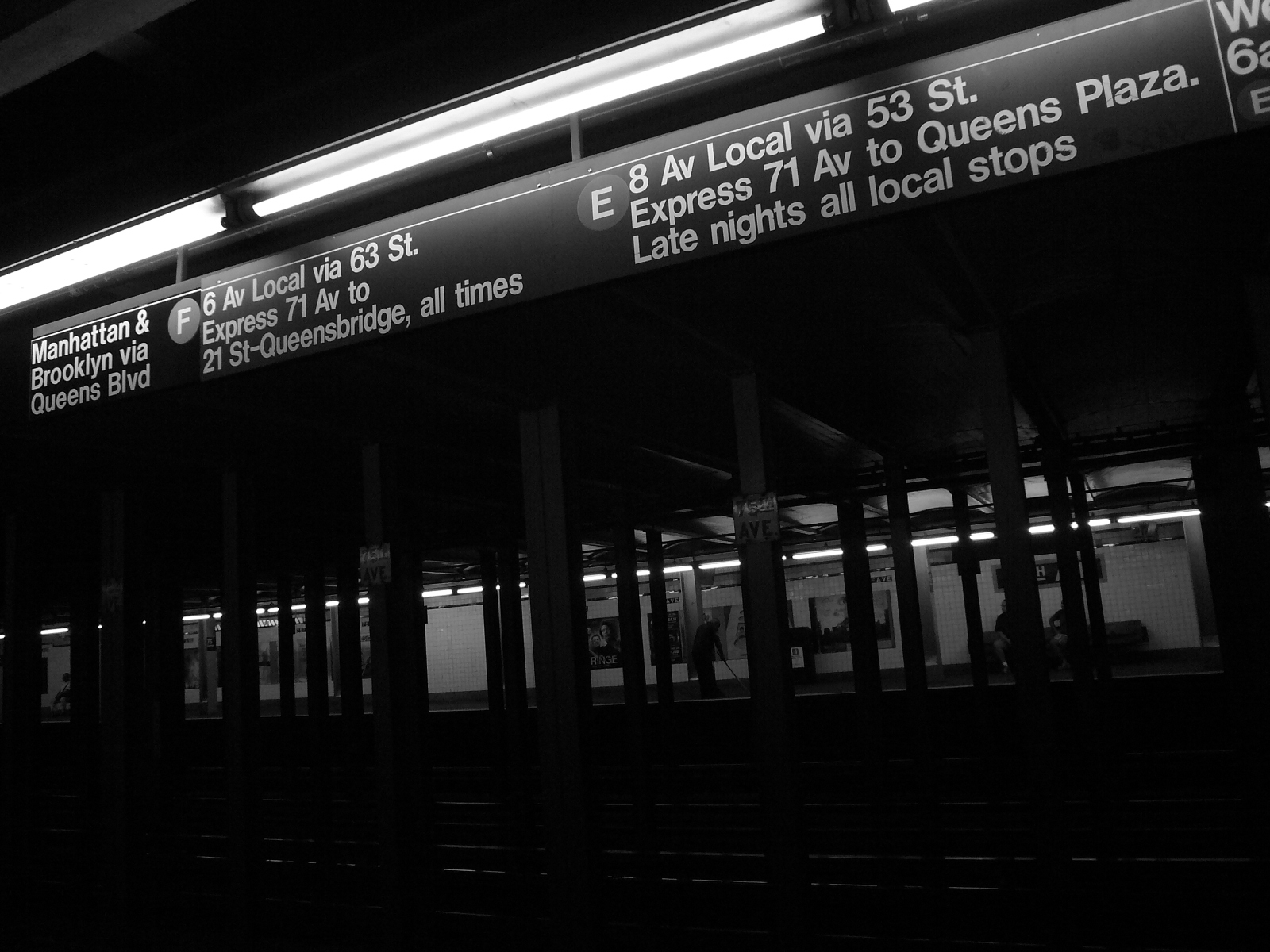In this black and white photograph, a late-night scene at a subway station unfolds, characterized by its dim, dingy ambiance and stark illumination from horizontal fluorescent lights. The setting is adorned with signs that provide critical transit information, indicating routes such as the E train, 8th Avenue local via 53rd Street, and late-night all local stops, as well as the F train, 6th Avenue local via 63rd Street, and express service from 71st Avenue to Queensbridge. The signs, positioned above the platform, convey essential directions, including routes through Manhattan and Brooklyn via Queens Boulevard. The station's structural elements, such as its pillars and white walls, are faintly visible under the harsh fluorescent glow, casting an eerie shadow reminiscent of a scene from a horror movie. Scattered throughout the platform are benches and a few isolated individuals, one possibly using a cane or a cleaning tool, emphasizing the platform's desolate and ghostly atmosphere. The vantage point of the photo captures a view across the subway tracks toward the far platform, where the sparsely populated scene unfolds in this stark interplay of light and shadow.